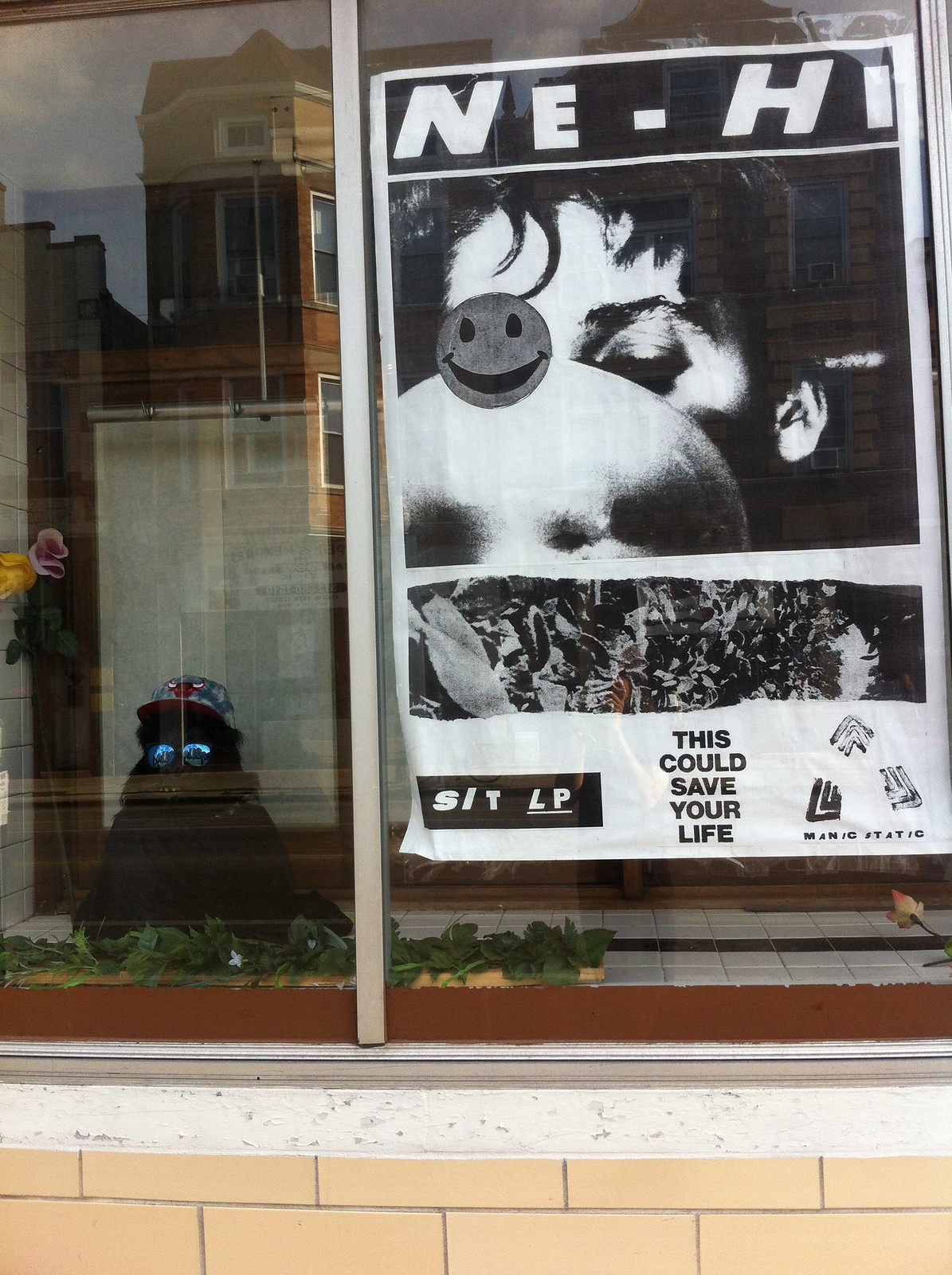The image depicts the exterior of a building with pink tile walls and white windowsills framing large glass windows. Reflected in the left glass window is a building across the street, while inside the window, partially obscured by surrounding foliage, is a fake animal or gorilla costume wearing sunglasses and a Chicago Bulls cap. The right side of the window features a large white paper poster, predominantly black and white, taped to the glass. At the top of the poster, a black bar contains the letters "NE-HI". Below this, there's a black and white photograph displaying part of a person's face with a round object and a smiley face superimposed over it. At the bottom of the poster is the text "This Could Save Your Life" alongside the letters "STLP" and a logo reading "Manic Static" on the bottom right corner.